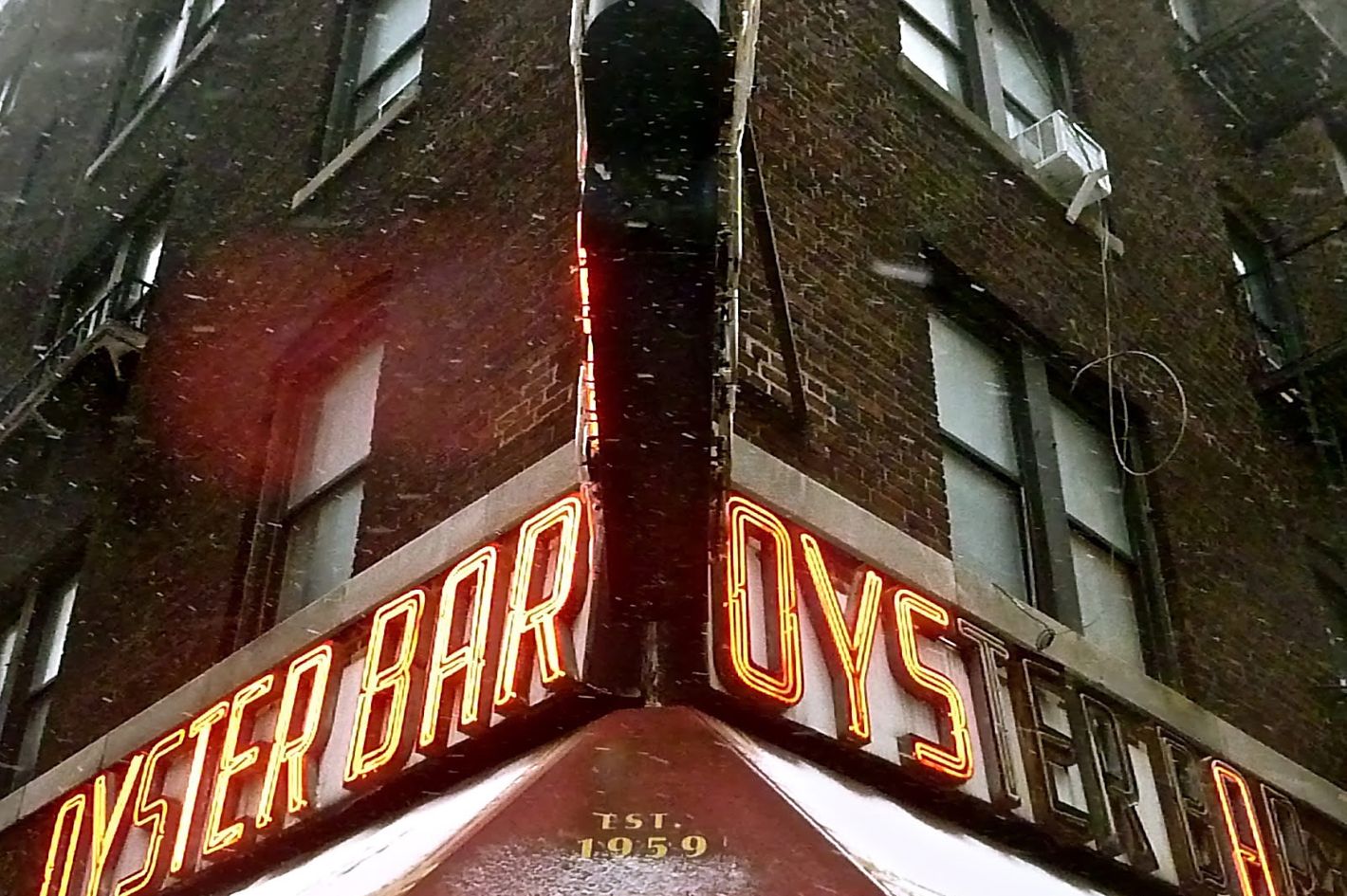This image captures a corner view of an old, two-story brick building characterized by a distinctive brownish-red hue. The building façade showcases a traditional brick pattern, with several windows adorning each story. Notably, the second story features an air conditioning window unit. Each side of the corner prominently displays a bright red sign that reads "Oyster Bar," although some letters (T, E, R, B, and the last R) are not illuminated. Situated below the sign on both sides, the inscription "EST 1959" can be seen. The picture is filtered with a bright red tint, enhancing the classic and nostalgic atmosphere of the scene. There is also a black section in the middle of the image, adding contrast to the vivid red filter.